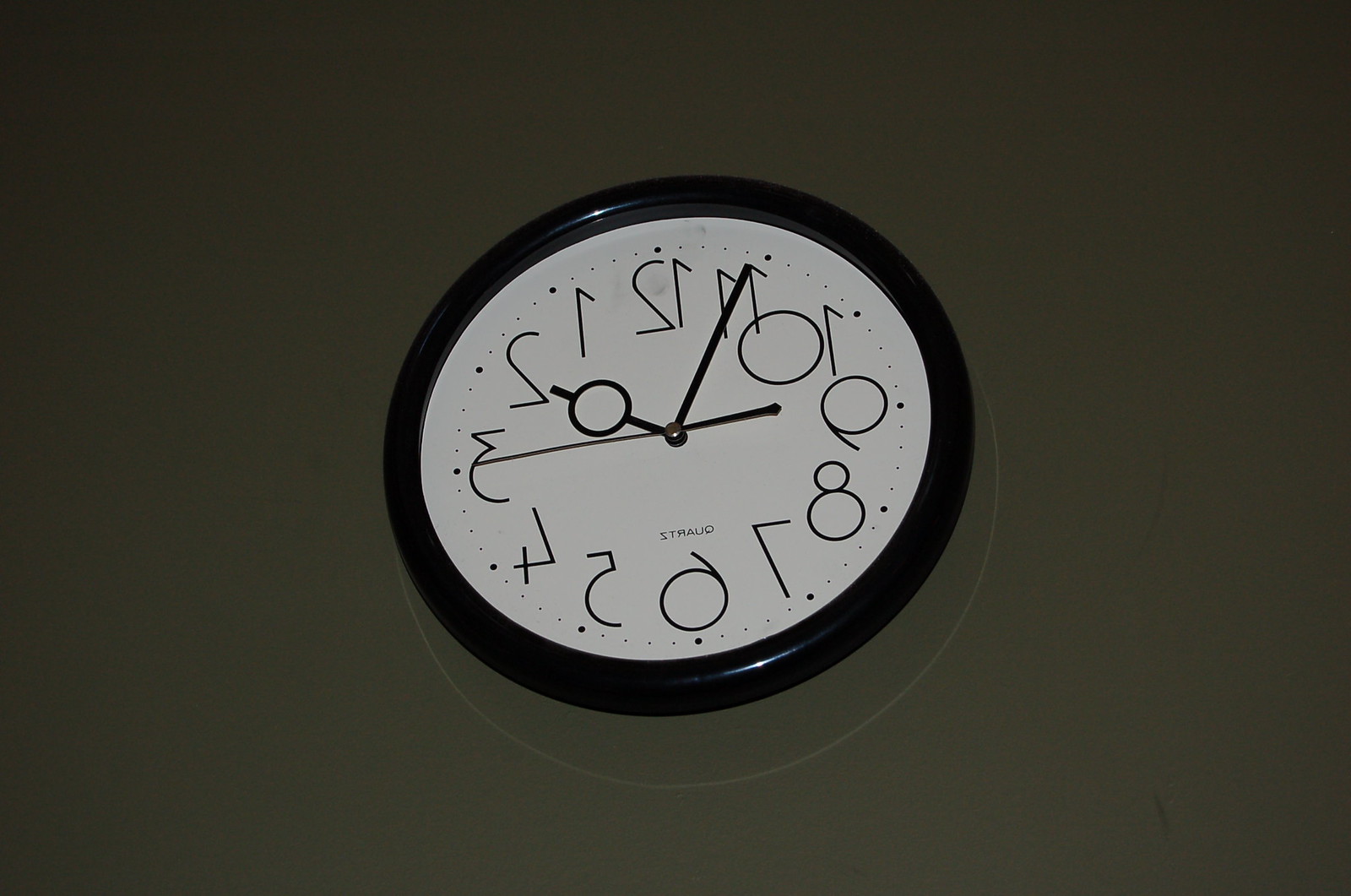This image features a uniquely designed clock set against a solid black background. The rectangular frame of the picture is slightly wider than it is tall, providing a balanced view of the centrally positioned clock. The clock itself is round with a thin, black border surrounding its white face. The black numerals on the clock face are printed in a reverse order, with '12' positioned at the top and the numbers proceeding counter-clockwise, culminating in a complete circle of reversed numerals. The digits are thin and elegant, emphasizing the clock’s distinctive design. The clock includes three black hands: an hour hand with an open circle near its tip, a matching black minute hand, and a long, slender second hand. The overall composition creates a striking contrast between the white clock face and the deep black background, highlighting the unusual numbering and the sleek design of the clock hands.